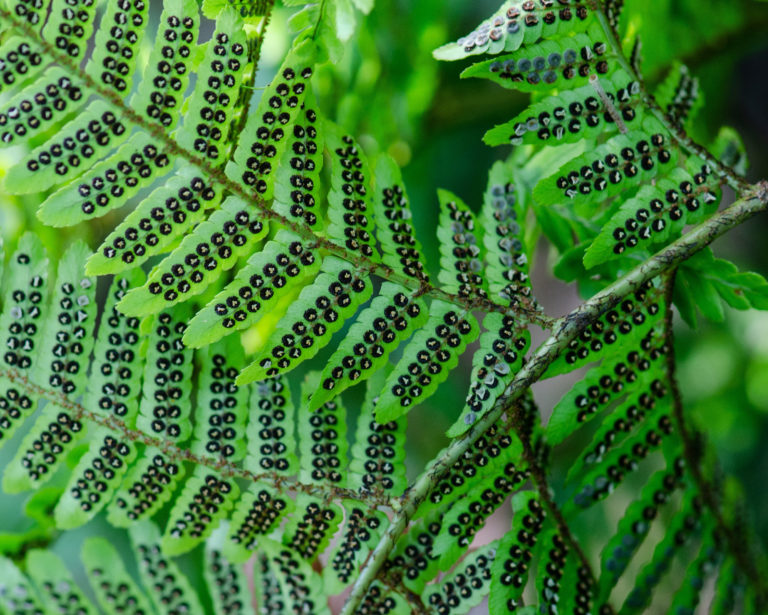This detailed outdoor photograph captures a close-up view of a vibrant green plant, taking up the entirety of the frame. The top portion of the image is fairly bright, with sunlight peeking through and casting a subtle glow, while the right half is slightly darker. A prominent skinny branch, green with some brown lines, enters from the upper right and extends towards the lower middle. Attached to this primary branch are multiple smaller stems, each hosting numerous leaves arranged symmetrically on either side. The top-left corner of the image is crisp, showcasing the intricate details of the leaves, while the bottom-right side becomes blurry, blending into the green backdrop of additional foliage.

Each leaf on the smaller branches is slightly pointed at the tip and adorned with unique black circular dots—approximately 7 to 12 per leaf—some dots featuring a delicate dashed pattern resembling gold. The uniform placement of these dots adds an interesting design aspect to the plant. Overall, the image provides a clear yet artistic representation of the leaf and branch structure, with a blurred green background hinting at more greenery beyond.